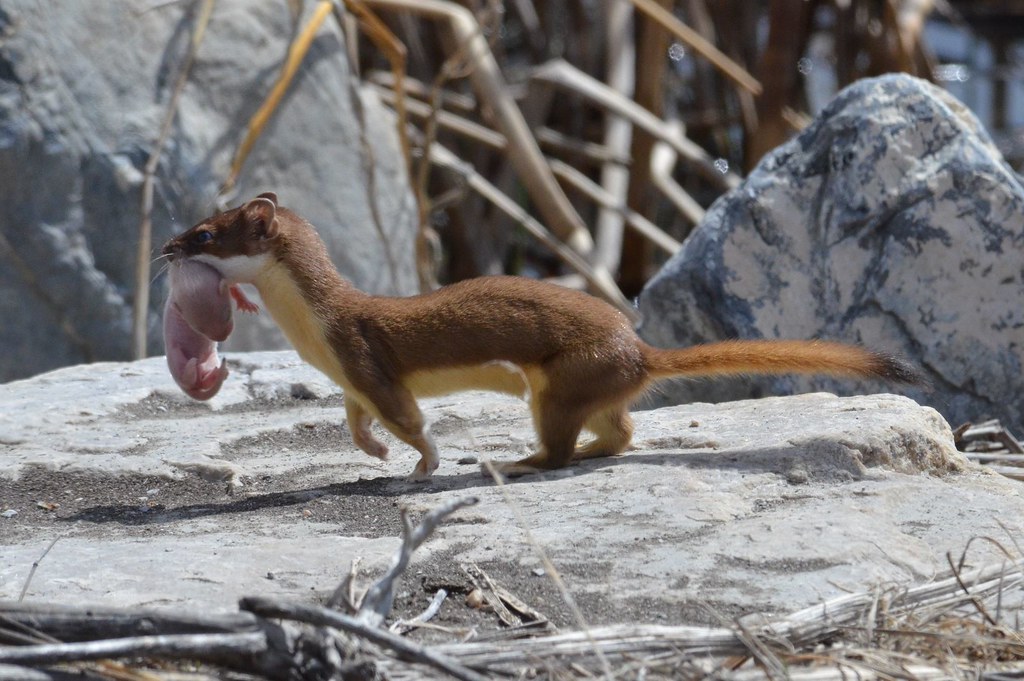In the center of the photograph, a brown and tan weasel with a white underbelly strides across a gray rock, carrying a very young, pink, and furless baby animal by the scruff of its neck. The baby animal, which could either be a recently born kit or a prey item such as a baby bird, dangles upside down from the weasel's mouth, its small tail clearly visible. The scene is framed by more rocks and a few branches, giving a somewhat barren appearance to the background. The weasel is alert and appears to be listening or looking toward something off to the left side of the photograph, its ears pulled back as if poised for action. The photograph captures a moment of movement and alertness in the wild, with the weasel's small but determined figure at the forefront.